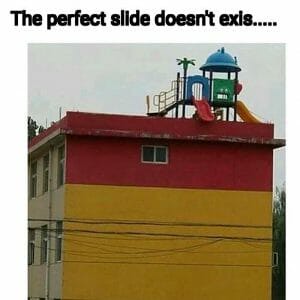This image humorously juxtaposes an ordinary children's playground with an absurdly dangerous setting. The black text at the top of the image reads, "The perfect slide doesn't exist....." on a white background that is not aligned with the photograph, creating a playful introduction to the scene. Showcased in the image is a tall, rectangular building with a flat roof. The building's facade is vividly painted, featuring a bright yellow bottom two-thirds and a dark red upper third, with a vertically split window visible on its side and additional windows on its front. Atop this building is a whimsical children's playground set made of plastic and metal, designed with stairs, platforms, and three slides: one shallow and brown, one red, and one orange. Each slide descends perilously off the edges of the rooftop, with the red slide dangerously extending over the edge of the building. The photo is taken on a gray, overcast day, further contributing to the surreal and precarious juxtaposition of a playground high above the ground.